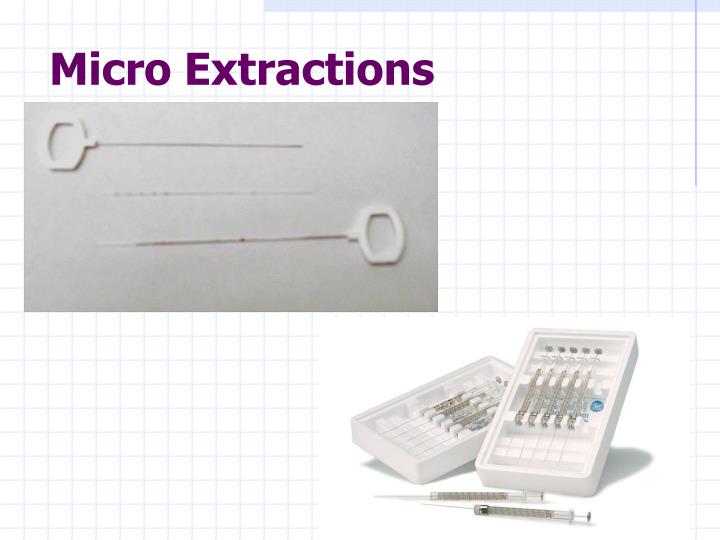Against a light blue checkered background, the title "Micro Extractions" is prominently displayed in plum purple text in the upper left corner. Below the title, there is a gray box containing three very long needles; the top and bottom needles have oval-shaped white plastic grips, while the center needle lacks a gripping device. In the bottom right corner, two rectangular plastic containers hold five needles each, secured in individual slots. Below these containers, two syringes are partially extended with their needles visibly protruding. Overall, the slide or page presents various tools and equipment used for micro extractions.